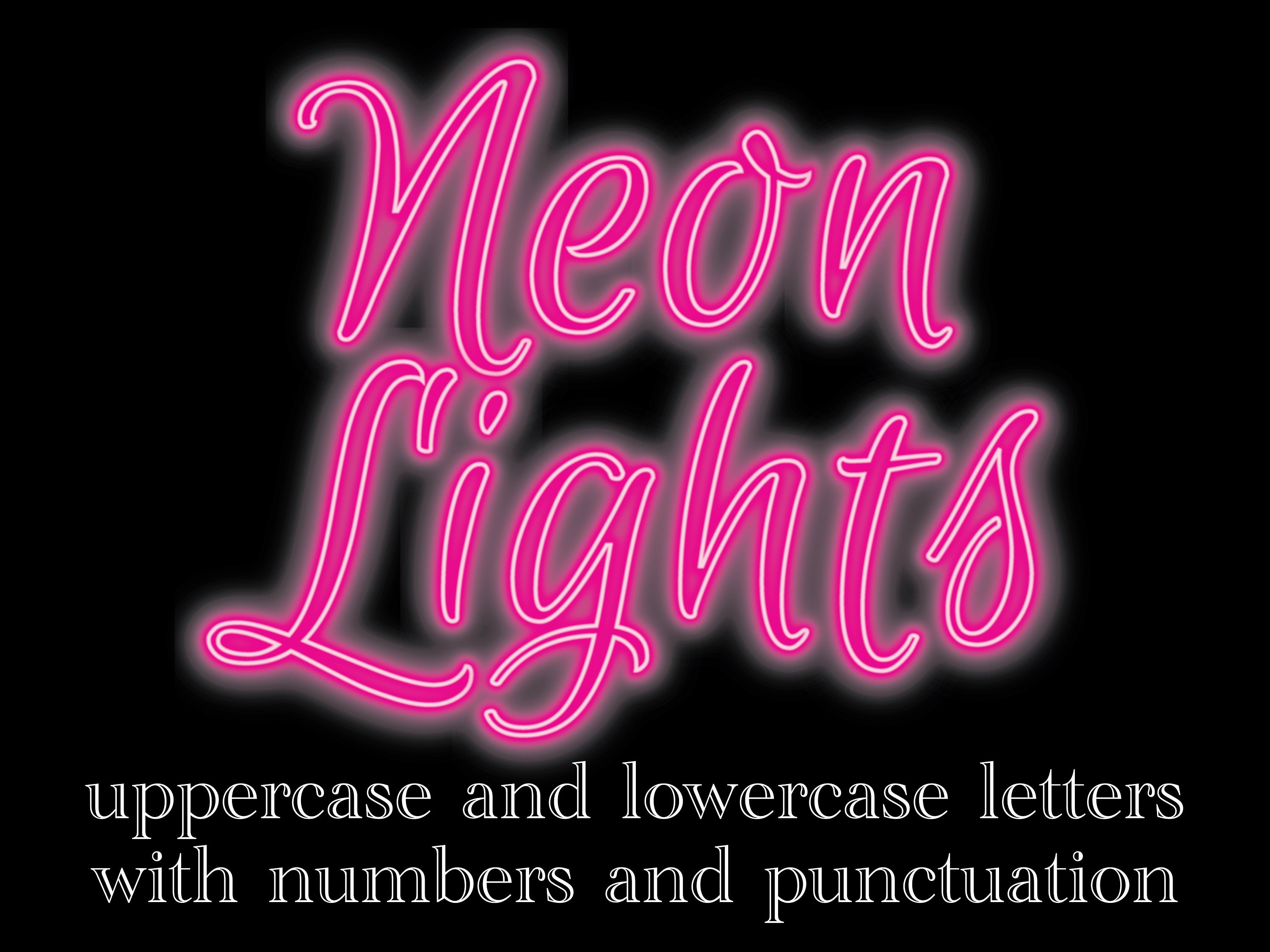This rectangular promotional image showcases a neon-style font on a pure black background. At the top and spanning the center, the words "NEON LIGHTS" are prominently displayed in a bright, vibrant pink color with a faint halo-like glow, mimicking the effect of actual neon lights. The text "NEON" is written in a slightly cursive style, with the capital "N" followed by lowercase "e," "o," and "n." Below it, the word "LIGHTS" follows a similar format with a capital "L" and lowercase "i," "g," "h," "t," "s." Occupying about two-thirds of the image, this neon text stands out with white outlines adding to the glowing effect. Beneath this, in a smaller, slightly 3D white lettering, the text reads "uppercase and lowercase letters with numbers and punctuation." The overall aesthetic gives a sense of digital artistry, possibly serving an advertising purpose, though the exact nature of what's being promoted remains unclear.